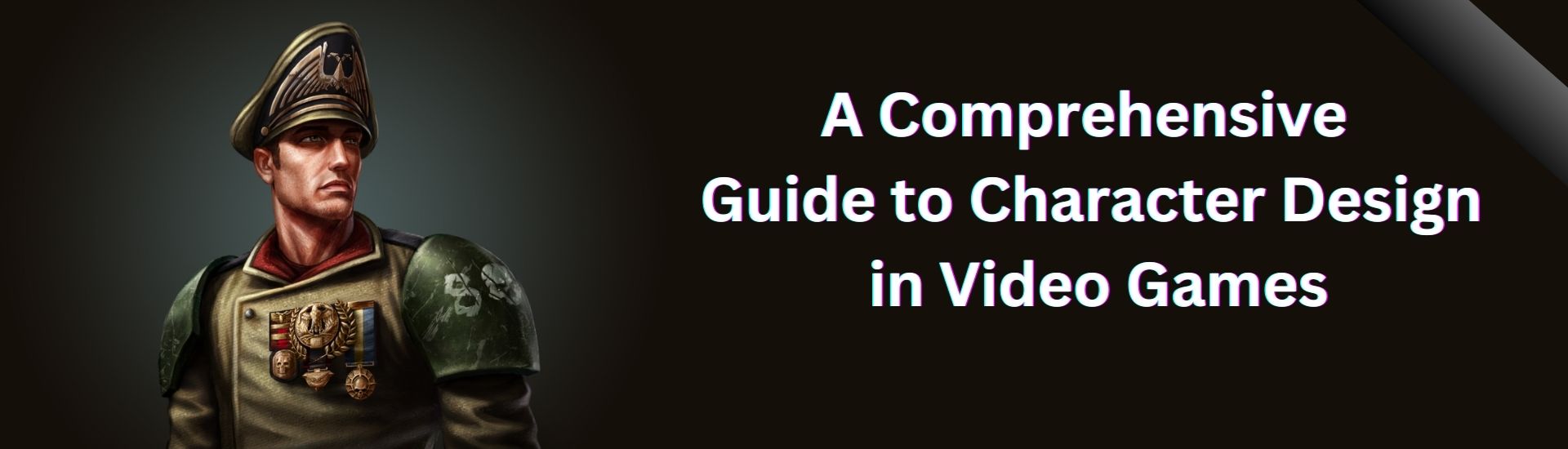The image features a detailed banner with a historical soldier prominently displayed on the left side. The soldier is dressed in a distinguished uniform, showcasing a gold-colored front adorned with approximately three to six medals on his chest. His shoulders and arms are covered in green metal-like armor, accented by white letters. His collar is red near his neck, fastened with a single button on the left side. The soldier, facing towards the right, wears a distinctive goldish helmet that slopes upwards at the front and tapers downward at the back, casting a shadow over his eyes but leaving his ear, nose, and frowning mouth visible. To the right of the soldier, white text reads: "A Comprehensive Guide to Character Design in Video Games." The background is a dark gray, with a dividing line in the upper right-hand corner separating the edge from the rest of the banner's design.